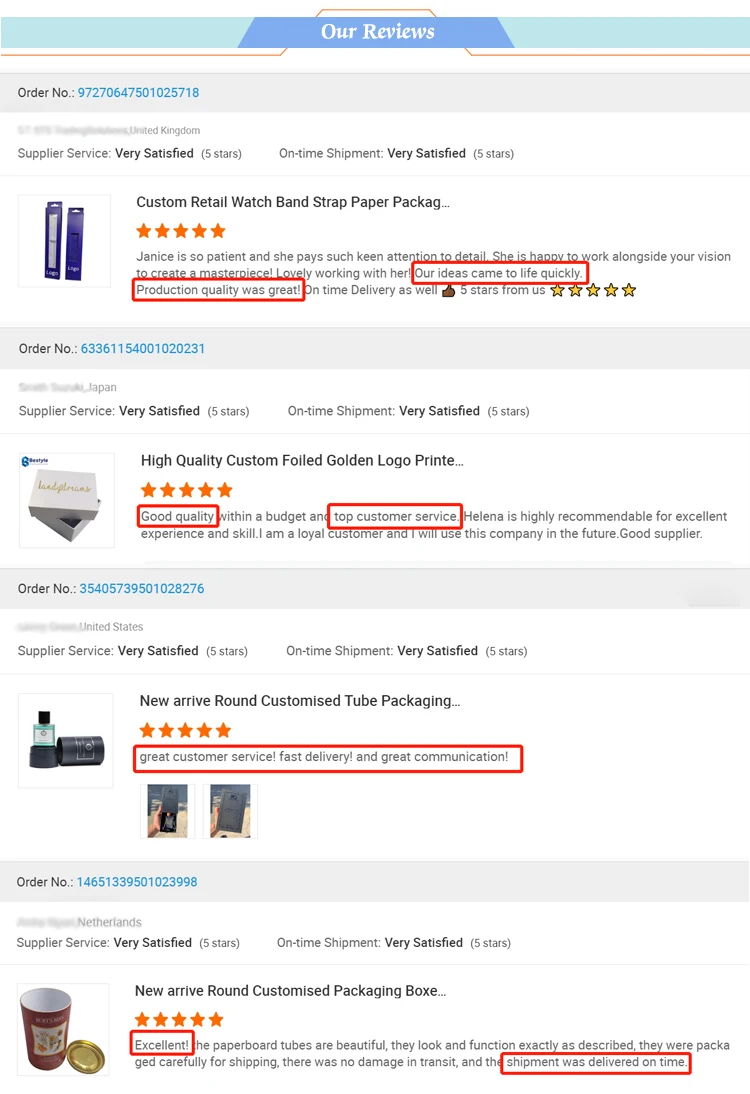This screenshot features a vertically oriented review summary with multiple rows, each detailing different customer reviews. At the top, a light blue stripe extends from the upper left to the upper right. Centered against it, on a darker blue stripe, is the text "Our Reviews."

The next row displays "Order Number" on a gray background, with the specific order number highlighted in blue. The creator of the screenshot has anonymized reviewers by whiting out their names but has left the countries visible.

1. **Reviewer from the United Kingdom**:
   - **Supplier Service**: Very satisfied (5 stars)
   - **On-time Shipment**: Very satisfied (5 stars)
   - **Product**: Custom retail watch band, strap, paper package
   - **Highlighted Comment**: "Our ideas came to life quickly. Production quality was great."

2. **Reviewer from Japan**:
   - **Supplier Service**: Very satisfied (5 stars)
   - **On-time Shipment**: Very satisfied (5 stars)
   - **Product**: High quality custom foiled golden logo
   - **Highlighted Comment**: "Good quality, top customer service."

3. **Reviewer from the United States**:
   - **Supplier Service**: Very satisfied (5 stars)
   - **On-time Shipment**: Very satisfied (5 stars)
   - **Highlighted Comment**: "Great customer service, fast delivery, and great communication."
   - Additionally, this reviewer has included images of themselves with the product.

4. **Bottom Review**:
   - **Highlighted Comments**: "Excellent" and "Shipment was delivered on time."

Each highlighted comment is bordered in red for emphasis, indicating the most noteworthy aspects of the reviews.